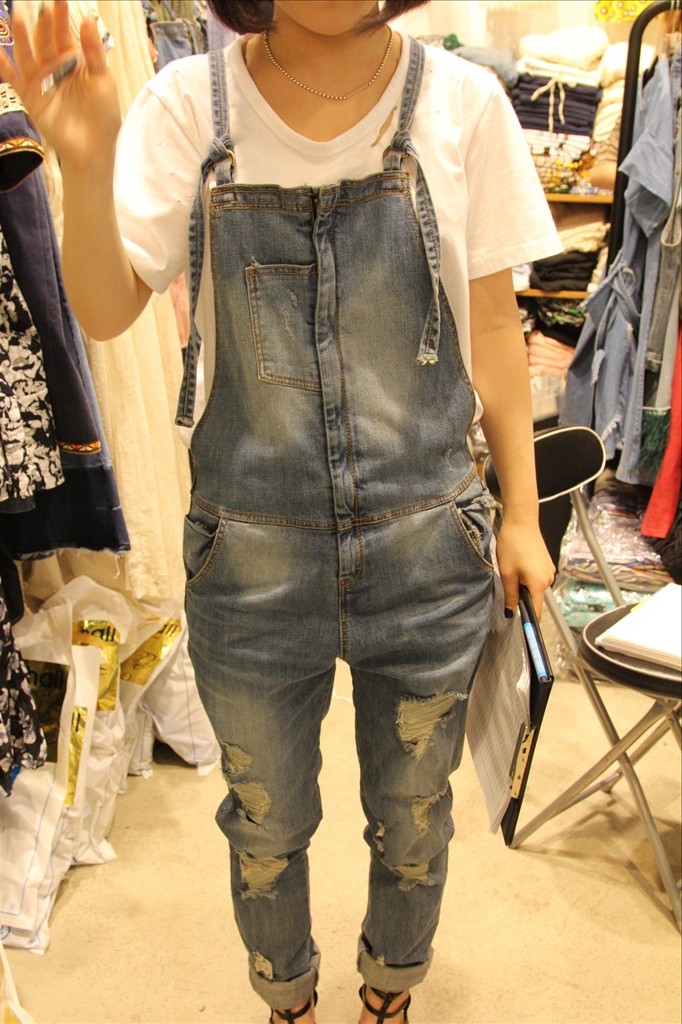The image depicts a young woman with a short bob hairstyle, characterized by chin-length dark brown hair. Her face is cropped out, revealing only her chin down to her ankles. She is dressed in oversized, baggy denim overalls that appear well-worn, particularly around the mid-thigh and down the front of the legs where the fabric is frayed and patched, giving a distressed look. These overalls have long, dangling straps and are cuffed at the bottom. She wears a plain white, slightly oversized V-neck T-shirt beneath the overalls, and a white beaded necklace adorns her neck.

In her left hand, she holds a black clipboard containing a stack of white papers and a pen. Her right hand gently holds a pencil between her index finger and thumb. On her feet, she wears a pair of casual heels, adding a slightly dressy touch to her otherwise laid-back outfit.

The background suggests she is in a clothing store or possibly a private, appointment-only boutique. Behind her are several wooden shelves filled with neatly folded clothes in various colors, stacked on three visible tiers. To her right, a black metal bar supports clothes hanging vertically from hangers, while more garments hang on unseen racks to her left. The flooring appears to be beige carpet or perhaps stone, though it's difficult to distinguish any specific pattern or texture. The environment is dense with clothing and general retail ambiance.